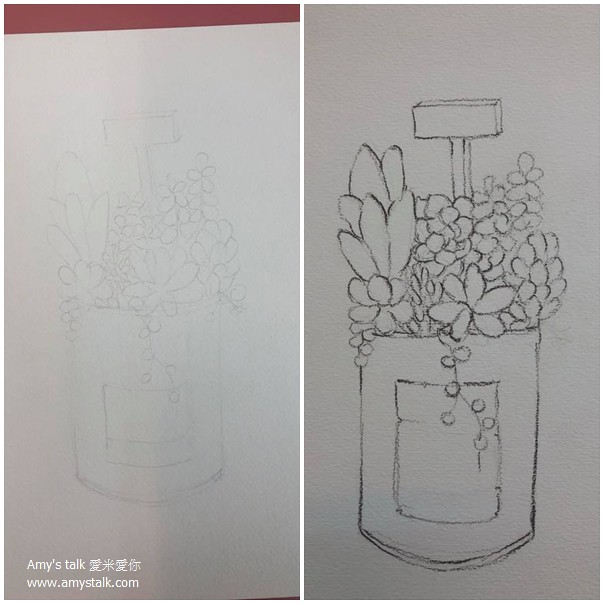This photograph showcases a pair of drawings placed side by side. The drawing on the left is slightly lighter compared to the one on the right, suggesting that the left might be an initial sketch, while the right is a more finalized version. Both drawings depict a cylindrical container, possibly a can or a flower pot, from which an array of succulents is growing. The succulents vary in height and form, with some tall and upright, and others draping vine-like in front of the container.

The medium used appears to be charcoal or a sketch pencil, giving the drawings a textured, classic look. Emerging from the succulent pot is a wooden stake, typically used to label plants, though it remains blank in this depiction.

In the bottom left corner of the drawings, the artist has signed with the name "Amy's Talk" along with a website, "www.amystalk.com," written in white. This adds a personal touch and directs viewers to more of the artist’s work.